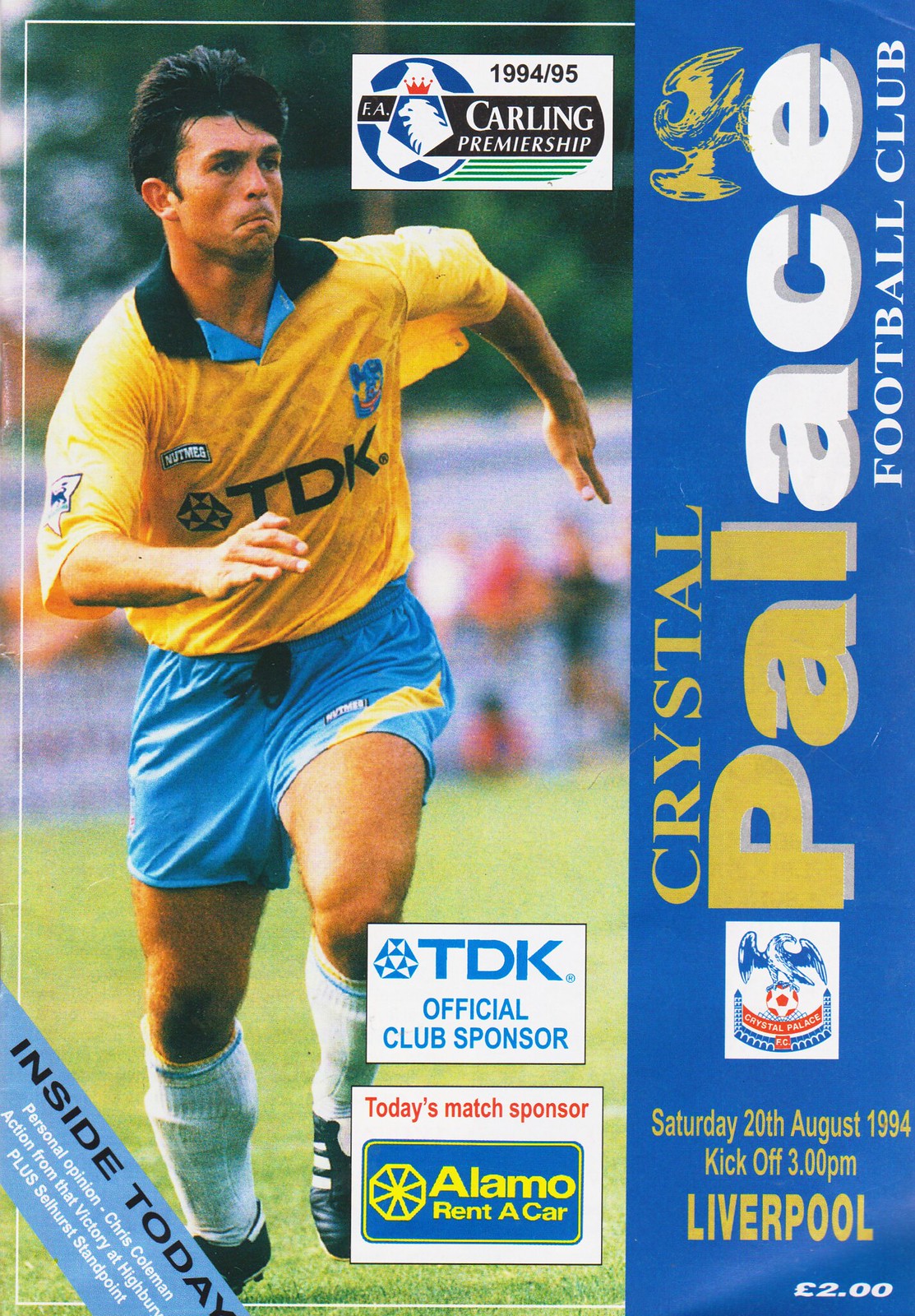The image appears to be a retro magazine cover featuring a dynamic action shot of a young Caucasian man with black hair, sprinting toward the viewer in a soccer uniform. He dons a yellow shirt, light blue shorts, high white soccer socks, and black cleats, racing across a blurred green field. The left two-thirds of the cover highlight this athlete, while the right third features vertically aligned text reading "Crystal Palace" in various shades of yellow and white, with the words "Football Club" beneath it. Additionally, a prominent club logo with an eagle symbol is placed near the top of the right side. At the bottom of the cover, horizontally oriented text announces "Saturday, 20th August 1994" with "Kickoff, 3 p.m." and "Liverpool" also featured. The cover price is marked at £2.00, and there are advertisements for Alamo Rent-A-Car and TDK, the club's official sponsor.